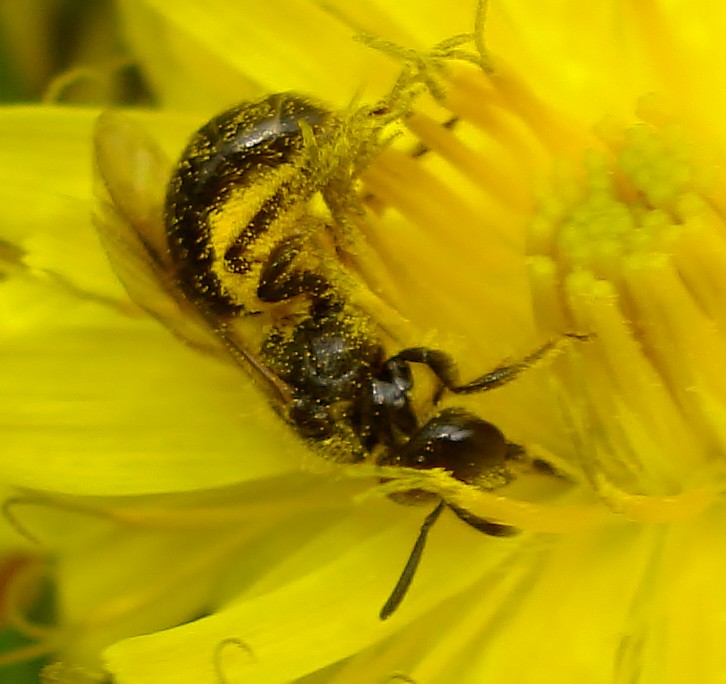This perfectly square image features a close-up of a yellow flower with many petals. Dominating the center is a bee, positioned upside down with its head facing downward and its tail and stinger pointing upward. The bee's black body is adorned with yellow stripes and is covered in numerous yellow pollen grains, especially on its legs and body. Its transparent wings, distinct antennae, and legs are clearly visible due to the extreme zoom. The background is filled with the blurred petals of the yellow flower, suggesting the bee is deeply engaged in gathering pollen. The very center of the flower has a slight greenish hue, adding contrast to the overall yellow ambiance of the image. The bee's detailed and intricate features stand out sharply against the soft, diffused backdrop of the flower's petals.